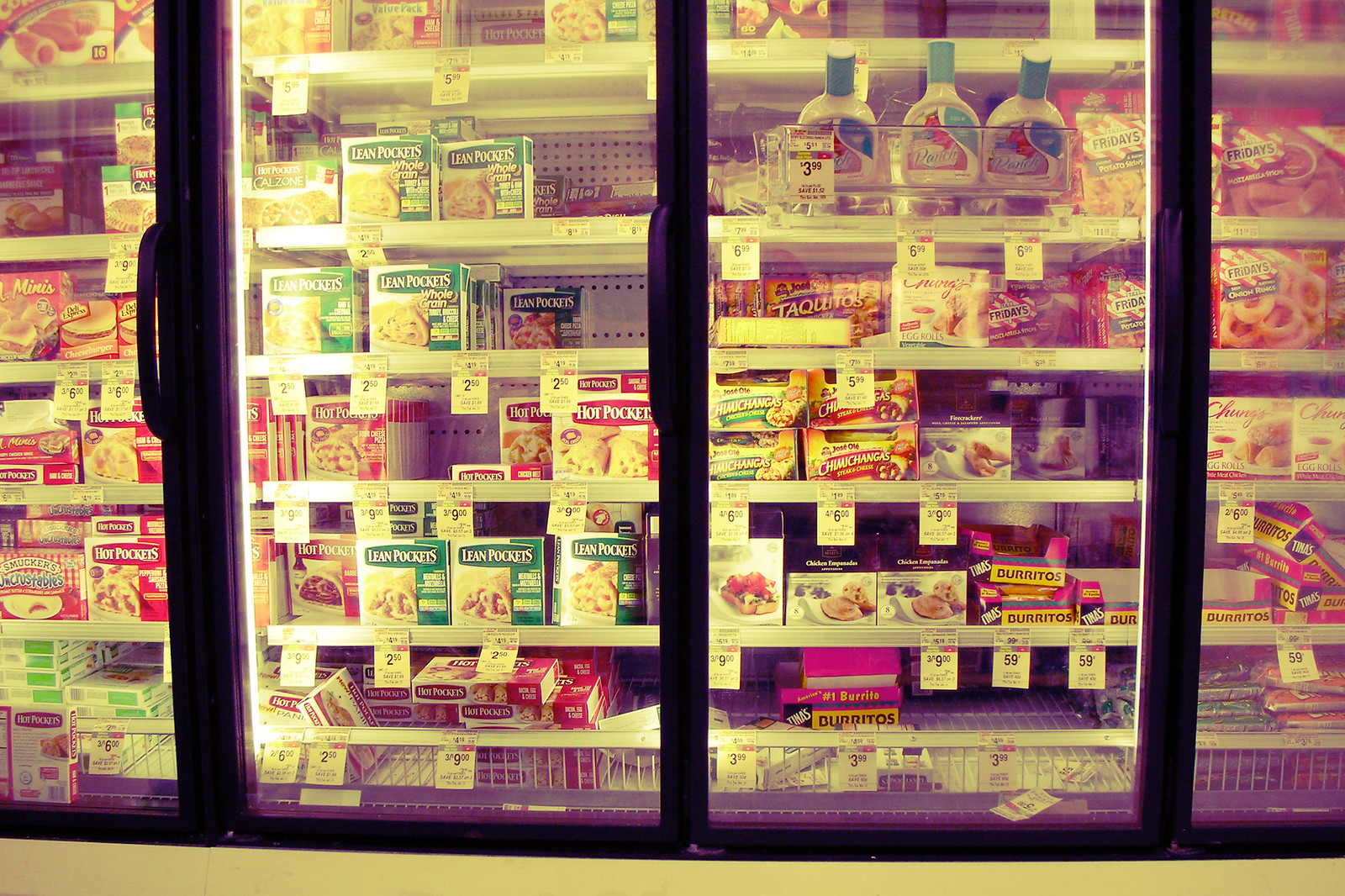This photograph captures a frozen food case in a supermarket, showcasing parts of four glass sections, each framed with a black border and featuring handles positioned at the right side middle of the doors. Inside the frosty display, multiple white shelves are neatly stocked with a variety of processed frozen food items and TV dinners. The shelves prominently feature products such as Lean Pockets, Hot Pockets, chimichangas, chicken empanadas, Tina's burritos, Smucker's Uncrustables, and TGI Fridays offerings like mozzarella sticks and onion rings. Price tags, including yellow "for sale" signs, are visibly attached to the shelves, highlighting discounts on select items. Additionally, a small plastic rack holding three bottles of ranch dressing hangs outside the third glass door on the right, located near the top. The assortment of frozen foods and the meticulously organized shelving dominate the entirety of the image, presenting a snapshot of a bustling supermarket's frozen aisle.